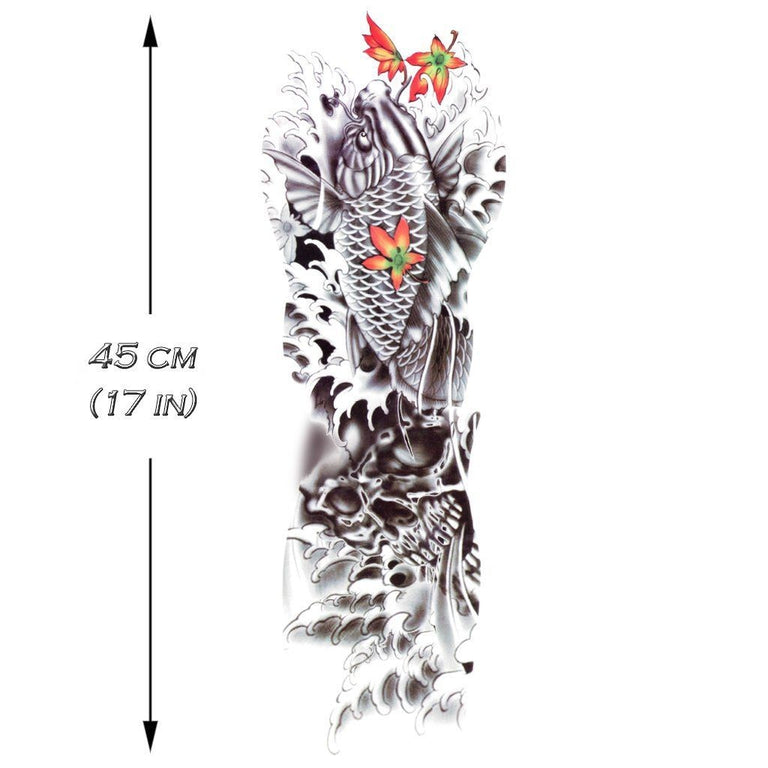This is an intricate rendering of a potential Japanese-style sleeve tattoo. The design predominantly features black and white shading, characterized by detailed depictions of a fish with outstretched fins, waves, and a skull subtly merging into the water patterns beneath the fish. The fish occupies the upper part of the image, pointing upward, while the skull, with discernible eye sockets, cheekbones, and teeth, is integrated into the lower part, partially obscured by the waves.

The tattoo's most notable color elements are three orange and green leaves or flower petals. These leaves flanking the fish resemble thick, holly-like leaves with orange exteriors and green centers. The complex texture around the fish and leaves evokes a snakeskin or honeycomb appearance, enhancing the design's visual depth.

On the left side of the tattoo, a vertical arrow indicates the potential size of the tattoo, marked as 45 centimeters (17 inches). This measurement suggests the piece could be conceptualized for a full sleeve tattoo. The overall design blends traditional Japanese motifs with modern artistic touches, making it a striking and detailed composition ideal for body art.